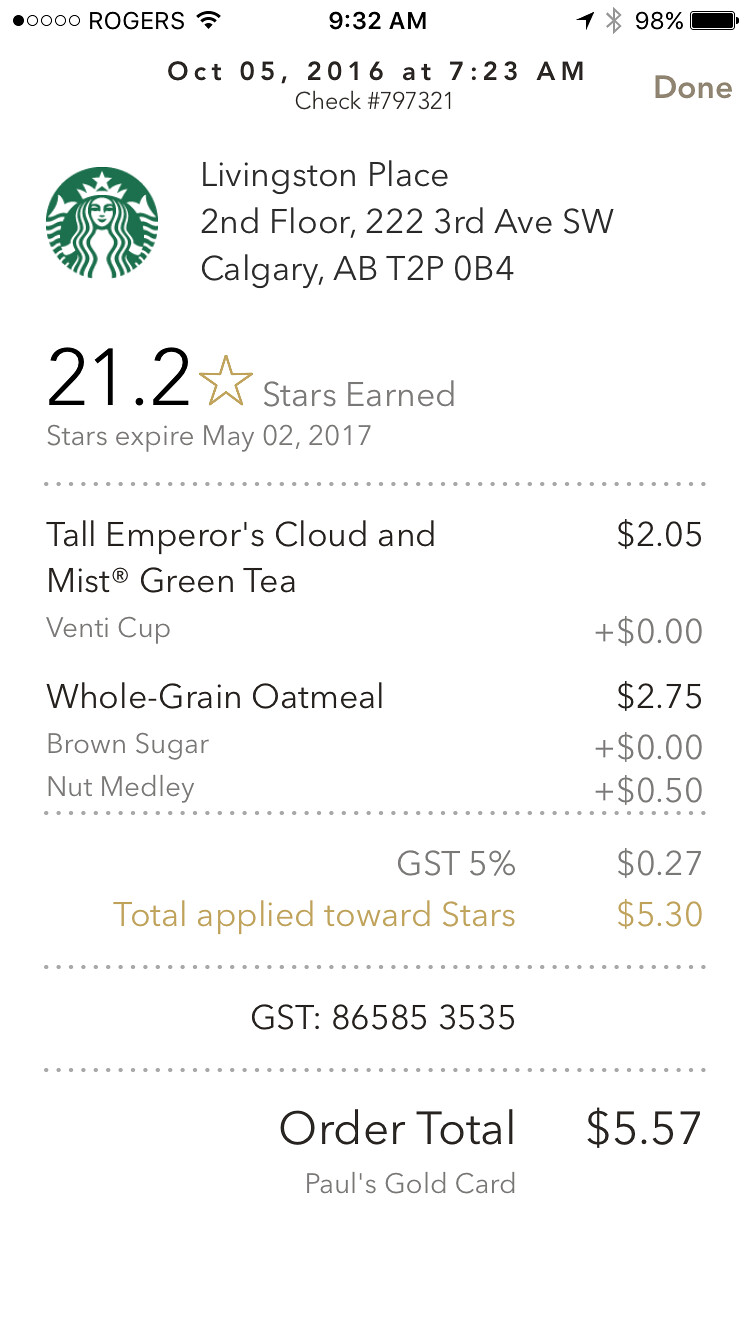The image is a digital receipt from Starbucks, screenshotted on an iPhone. The top left of the screen shows the ROGERS network with one out of five bars filled, indicating weak signal strength. Adjacent to this, the time reads 9:32 AM. On the top right, there's a black location icon, a grayed-out Bluetooth icon, and a battery status showing 98%.

The receipt is dated October 5, 2016, at 7:23 AM. It references a purchase at Starbucks located at Livingston Place, Second Floor, 222 3rd Avenue SW, Calgary, AB, T2P 0B4. The check number is 797321. The receipt details a purchase of a Tall Emperor's Cloud and Mist Green Tea for $2.05 and a whole grain oatmeal with added brown sugar ($0) and a nut medley ($0.50), totaling $2.75. With a 5% GST of $0.27, the total amount paid was $5.57, of which $5.30 was applicable towards the Starbucks loyalty program stars. The receipt notes the user's star balance as 21.2 stars, with an expiration date of May 2, 2017. The text detailing the amount applied towards stars is in brown, while the rest is in black. The receipt concludes with the mention of "Paul's Gold Card," indicating the loyal customer's membership status.